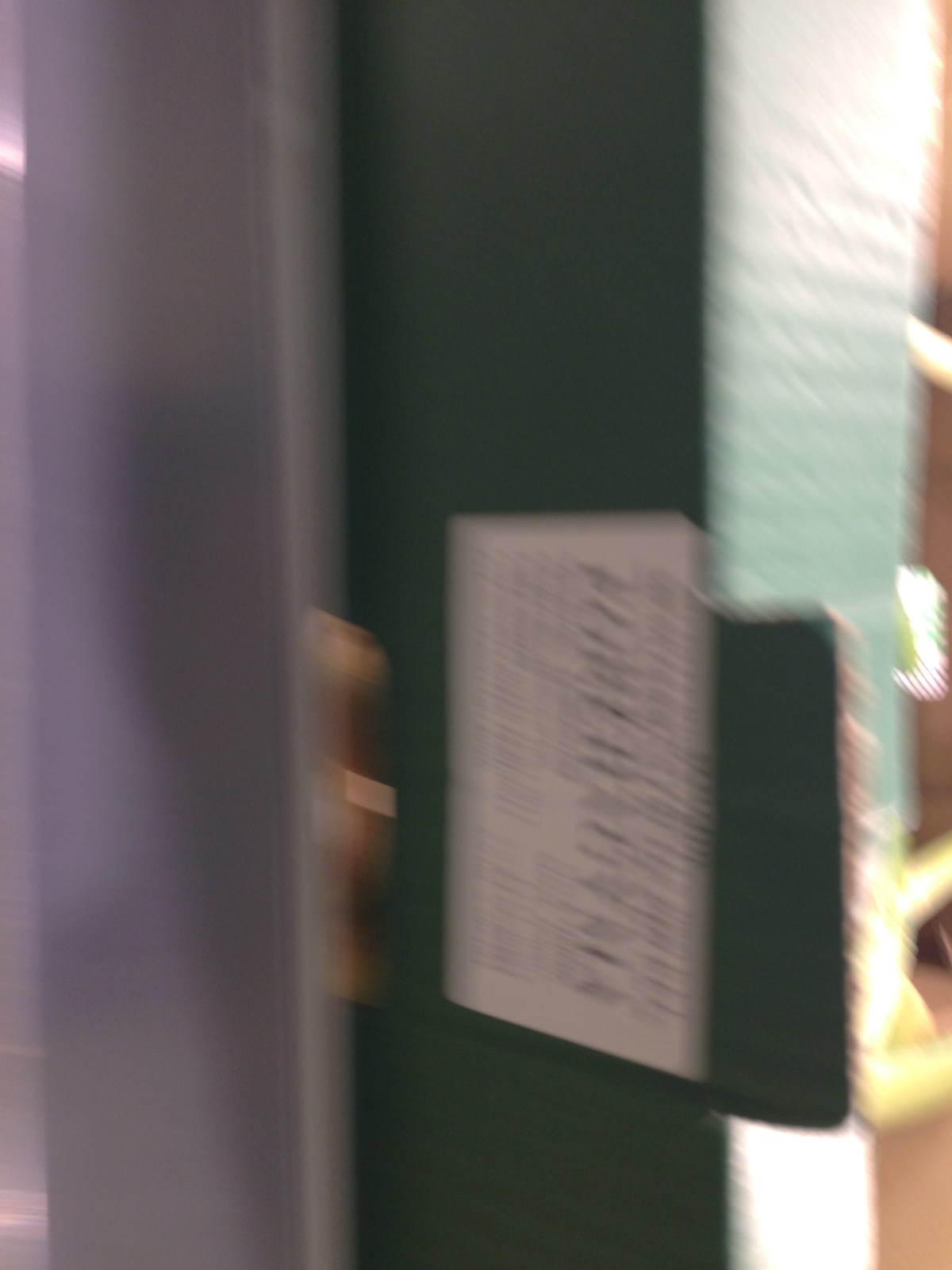The image is a blurred photograph, seemingly taken on its side. It depicts a rectangular cardboard box placed diagonally, with one side of the box oriented toward the top of the photograph and the opposite side directed toward the center bottom. Due to the blurriness, the details of the contents, label, barcode, and item description on the box are indiscernible. The box itself appears to be dark forest green, featuring a white label with black writing on its front. The photograph seems to have been taken on a gray or off-white table within a room. There's a possibility of a brown-colored table visible in the far background, adding depth to the image.